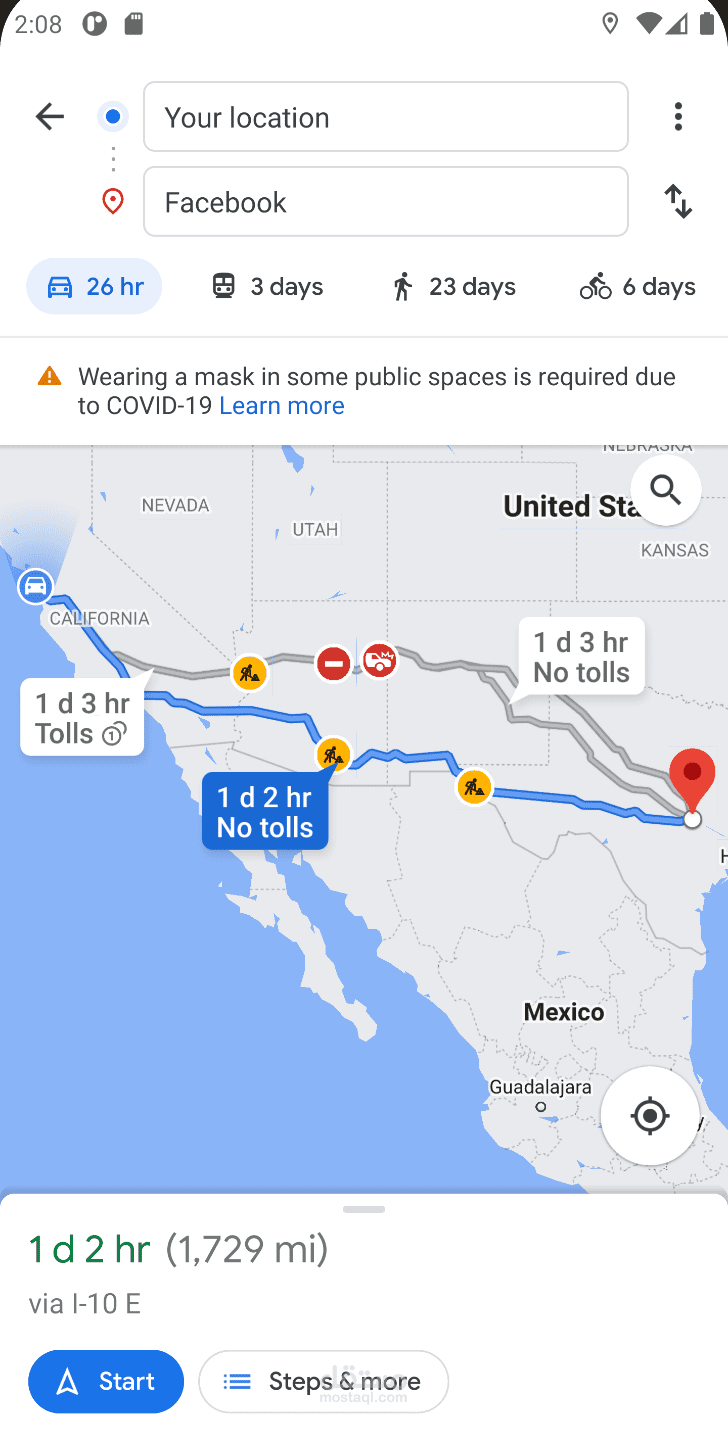This is a detailed screenshot of a navigation screen, likely from Google Maps, providing comprehensive travel information for a planned route. 

At the top of the image, several icons are present, including a circular disc, a location pin, Wi-Fi signal, and battery status, alongside the number "208". Below this header, a black back arrow is visible, and a blue circle icon is prominently displayed. The screen shows two distinctive boxes: one labeled "your location" with three gray dots, and another labeled "Facebook" with two arrows and a red location pin icon.

Moving further down, a series of icons and travel estimates are displayed. A car icon notes a travel time of 26 hours in blue text. A tram icon indicates a travel duration of three days, a walking icon suggests 23 days, and a bike icon marks six days. Additionally, there is an advisory message with an orange triangle indicating, “Wearing a mask in some public spaces is required due to COVID-19,” followed by a "Learn more" link in a blue box.

A detailed U.S. map in gray occupies the central part of the screen, showcasing regions including Mexico, California, Nevada, Utah, and Kansas. The map includes blue and gray route lines, gold icons, and red icons. Notably, near Mexico, a white circle with a gray bullseye is visible, and by Texas, a red location pin stands out. Overlaying the map is a white box indicating "one day, three hours, no toll."

Descending the image, additional travel details are listed. One blue box specifies "one day, two hours, no tolls," while another white box states "one day, three hours, tolls." A blue and white car icon appears near California.

At the bottom, the estimated travel time is highlighted in green as "one day, two hours," coupled with a gray note of "1,729 miles" and the via route "I-10 East." Navigation options include a blue and white "Start" button and a gray, white, and blue "Steps and more" button.

The entire screen is a detailed portrayal of a user’s navigation plan, filled with icons, advisories, and extensive route information, all encapsulated within a user-friendly interface.